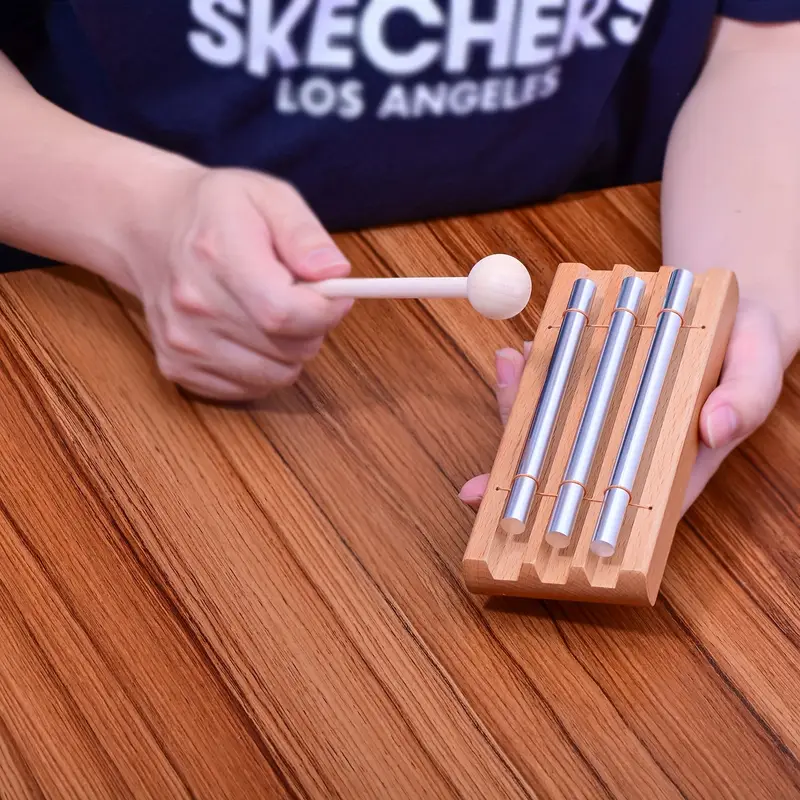This image depicts a Caucasian woman demonstrating a unique musical instrument atop a beautifully grained wooden table. The instrument itself is a small, rectangular wooden block with three longitudinal cutouts. Attached to these cutouts are three metallic rods of varying lengths, presumably designed to produce different tones when struck. The woman, wearing a navy blue T-shirt with "Skechers" in bold capitals and "Los Angeles" beneath, holds a white wooden mallet in her right hand. This mallet, resembling a lollipop with its knobbed end, is poised above the metallic rods, suggesting the instrument is played by tapping the mallet on the rods to produce sounds. Her left hand supports the darker wooden block. Although the exact name and sound of the instrument are unclear, the arrangement and elements imply its function in creating musical notes.